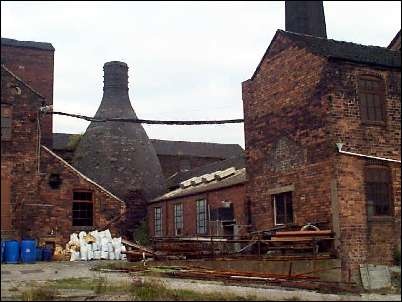This photograph captures an aged, industrial complex with red and brown brick buildings, possibly a few centuries old, viewed from across a street. The landscape-format image, though low in resolution, vividly depicts the character and details of the site. To the right side, there's a prominent two-story building, alongside various smaller structures, with one noticeable black roof and brown-paned windows. A tall chimney rises above this area. Another notable feature is the unique, kiln-like building towards the middle left, constructed of gray brick and resembling a fat wine bottle with a narrow neck and wide base; it even has a door at the bottom. The foreground includes a patch of scrubby grass, some concrete, and fencing, juxtaposed with blue recycling barrels and large white sacks near the left-side buildings. A white, overcast sky forms the backdrop, suggesting a serene, yet slightly desolate ambiance around the seemingly abandoned facility.